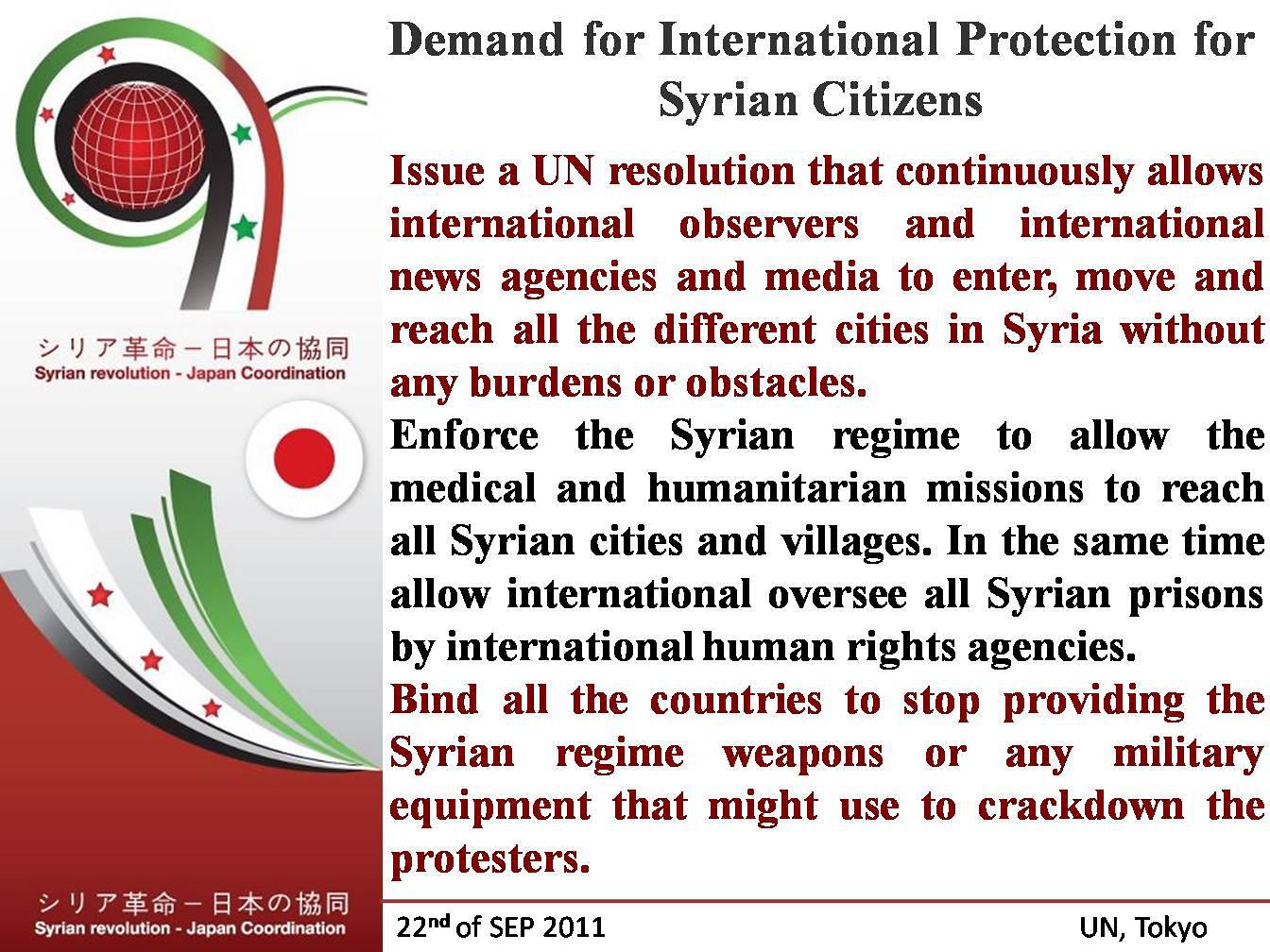The image depicts an advertisement for the Syrian Revolution Japan Coordination Meeting, held on September 22, 2011, at the UN in Tokyo. This event focuses on the demand for international protection for Syrian citizens. The left side of the image features a red, white, green, and gray color scheme, with a prominent red circle outlined in white, reminiscent of the Japanese flag. The right side of the image contains a significant amount of text in black and red, emphasizing key points. The text calls for a UN resolution to allow continuous access for international observers, news agencies, and media to enter and operate freely in Syria. It urges the overcoming of obstacles to enable medical and humanitarian missions to reach all Syrian cities and villages. Additionally, it demands international oversight of Syrian prisons by human rights agencies and calls for a binding cessation of military support to the Syrian regime to prevent the crackdown on protesters.